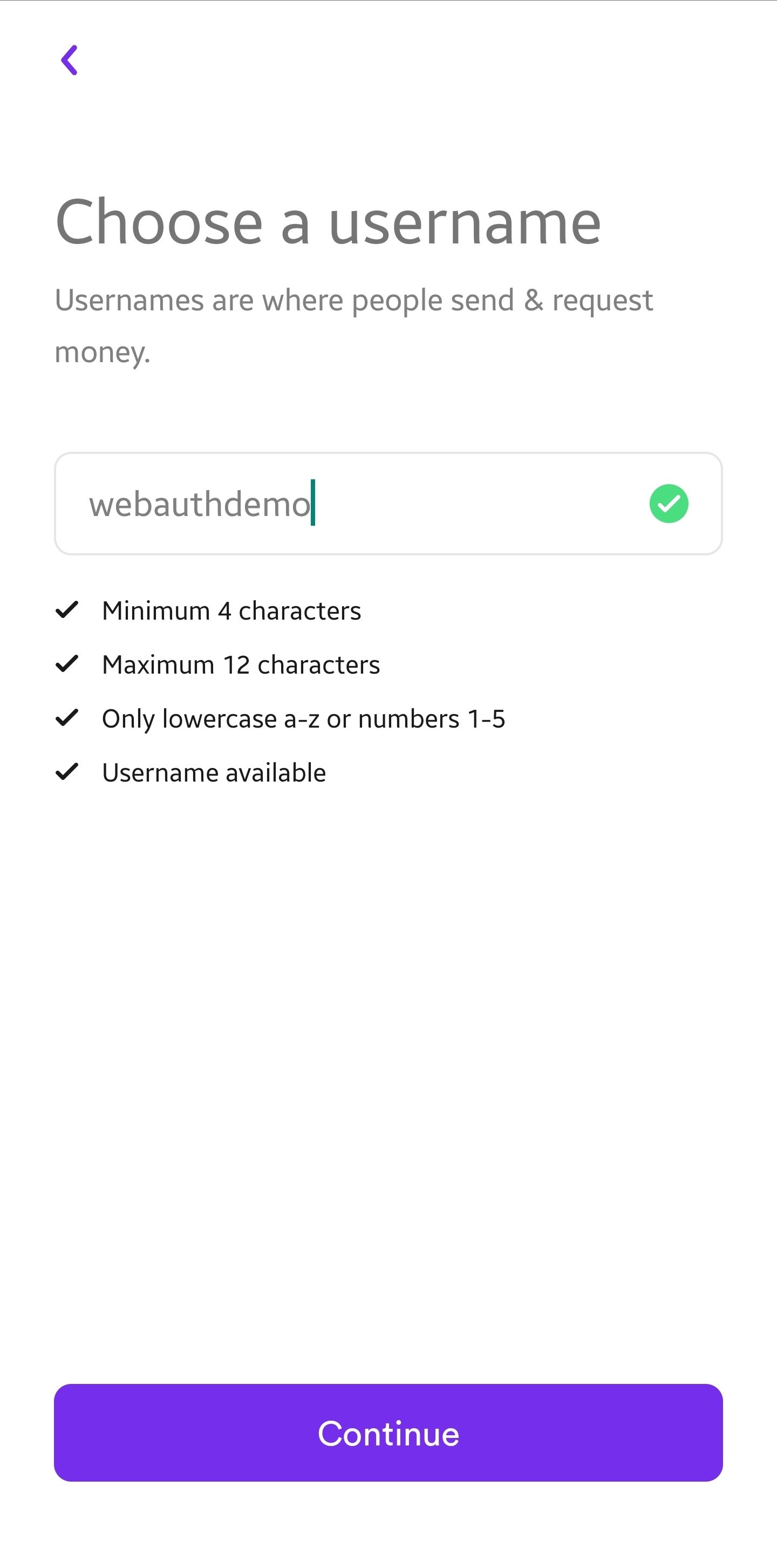This is a screenshot from a mobile application on a white background. At the very top, there is a backward arrow icon. Below it, in bold black font, are the words "Choose a Username." Beneath this header is an explanatory sentence indicating that usernames are used for sending and requesting money. 

Following this, there is a text box where the user can type in their desired username. Under the text box is a list of requirements that the username must meet: it should have a minimum of four characters and a maximum of twelve characters, contain only lowercase letters (a-z) or numbers (1-5), and be available for use. 

In this example, the username "WebAuthDemo" is typed into the text box. It meets all the specified criteria, as indicated by green checkmarks next to each requirement and a green checkmark within the text box itself, signifying that the username is valid and available.

After a considerable amount of white space, around two to three inches, there is a rectangular button that spans the entire width of the mobile screen. This button is labeled "Continue," prompting the user to proceed with their selected username.